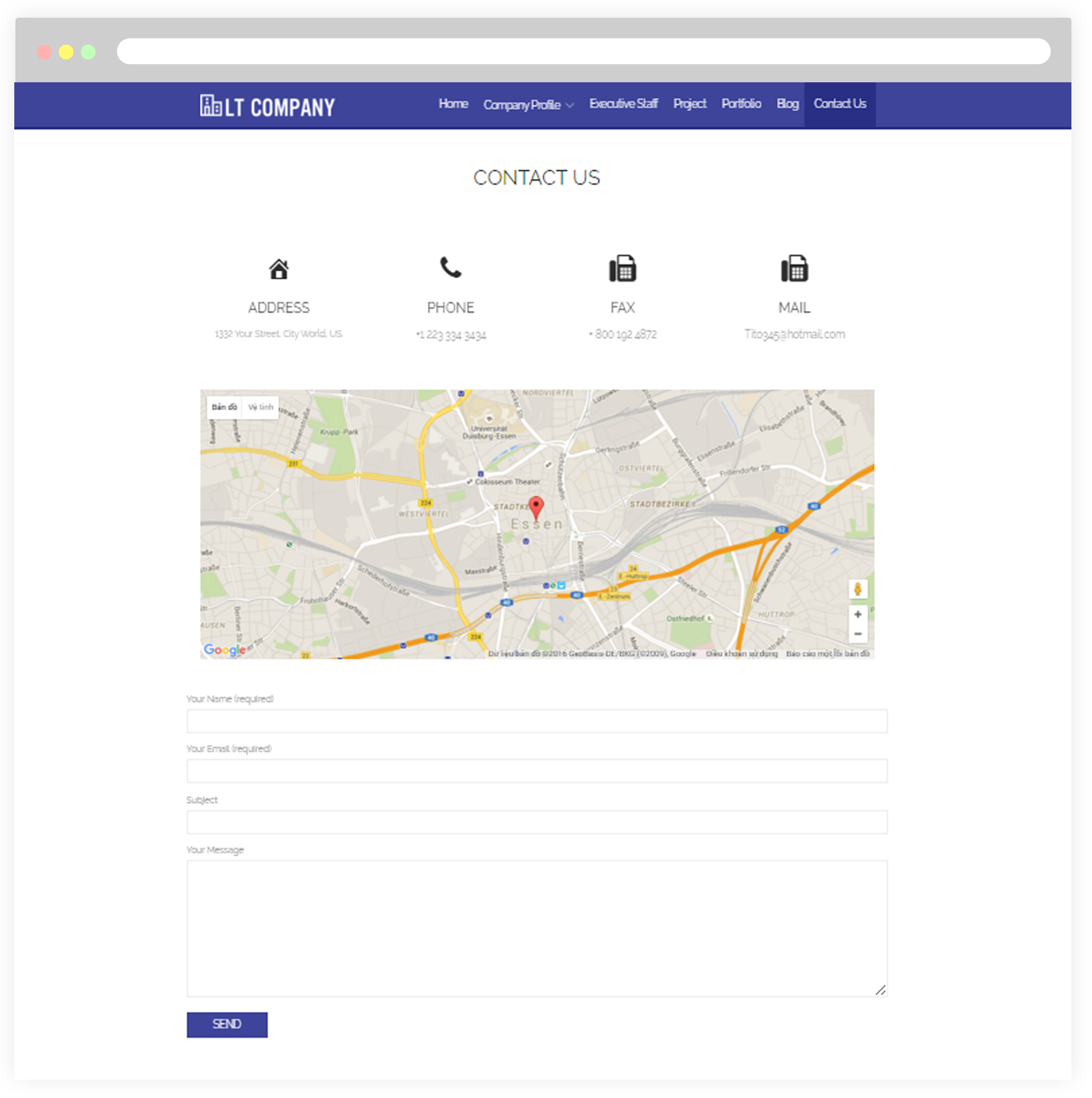The top of the webpage features a gray navigation bar with a white search bar inset, accompanied by three traffic light icons—red, yellow, and green. Below this, there is a blue rectangular section marking the start of the webpage, which prominently displays the LT Company logo and navigation menu in white text against a royal blue background. The logo consists of graphics of a tall building and a smaller building.

The navigation menu includes the following options: Home, Company Profile (with a dropdown menu), Executive Staff, Projects, Portfolio, Blog, and Contact Us. The "Contact Us" page is currently highlighted in a darker shade of blue, signifying the active section.

On the "Contact Us" page, contact information is provided in a structured layout. There is an icon of a house labeled "Address," with the placeholder text "Your Street, Your City, World, USA." Below this is a phone number, "1-223-334-3434," accompanied by a phone icon. Next is a fax number, "800-192-4872," beside an icon of a fax machine. Additionally, an email address "Tito 3459, or Tito 3453 @ Hotmail.com" is listed, accompanied by a mail icon.

In the center of the page, a map with a pin indicating a location labeled "S-N-E-S-S-E-N" is displayed, though the text is quite small and difficult to read. Below the map, a contact form is provided with fields for "Your Name (Required)," "Your Email (Required)," "Subject," and "Message." Users can fill in these details and press the blue "Send" button to submit their inquiries to LT Company.